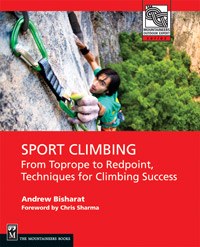This image depicts the cover of a sport climbing textbook. The top third of the cover showcases a bird's eye view of a man with dark hair climbing a nearly vertical, gray and brown rock face. Dressed in a green shirt, he reaches with his left arm to grasp a green metal clip embedded into the rock, while his right hand clings to the rock itself. Below him, a dense forest is visible, emphasizing the height of his climb. The background of the cover is predominantly red, and the text, all in white, includes the book's title, "Sport Climbing: From Top Rope to Redpoint - Techniques for Climbing Success," authored by Andrew Bisharat, with a foreword by Chris Sharma. In the bottom left corner of the cover, there's a logo and some text within a black box, though it's too small to read. The overall design of the cover combines striking visuals with informative text to engage readers and climbers alike.